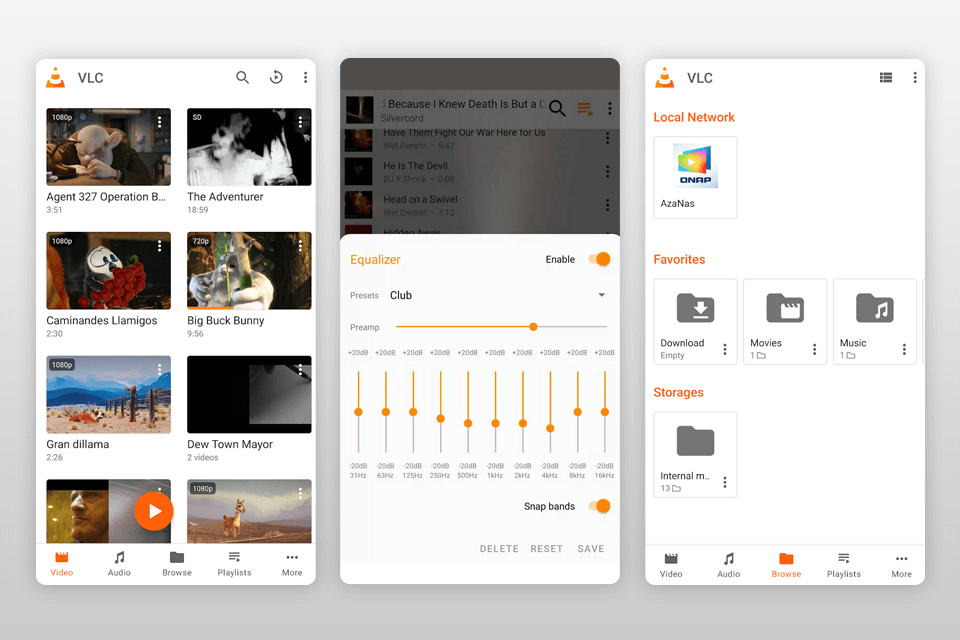The image resembles a collage of various multimedia elements and settings from different sources. At the top left, there are icons for VLC media player, a magnifying glass, a refresh button, and a menu symbolized by three dots. Below these icons, there's text labeling different videos: "Agent 327, Operation B, The Adventurer," followed by "Caminares Amigos" (2 or 3 episodes), and "Big Buck Bunny."

Prominent images include scenes from animations such as "Scranton Lava" and "Dude Town Mayor." Toward the bottom left, a face is depicted alongside an orange button. The lower section of the image features buttons labeled "Video," "Audio," "Browse," "Playlists," and "More."

Further descriptions include an equalizer panel with labels like "Club," "Preamp," "Enable," and frequency adjustments ranging from "131 kHz" to "8,000 kHz," with corresponding gain values. Specific adjustments like "+20 dB" are seen. Additionally, there are options to "Delete," "Reset," and "Save" configurations, with an identifiable unlock and release music button visible to the right side of the image.